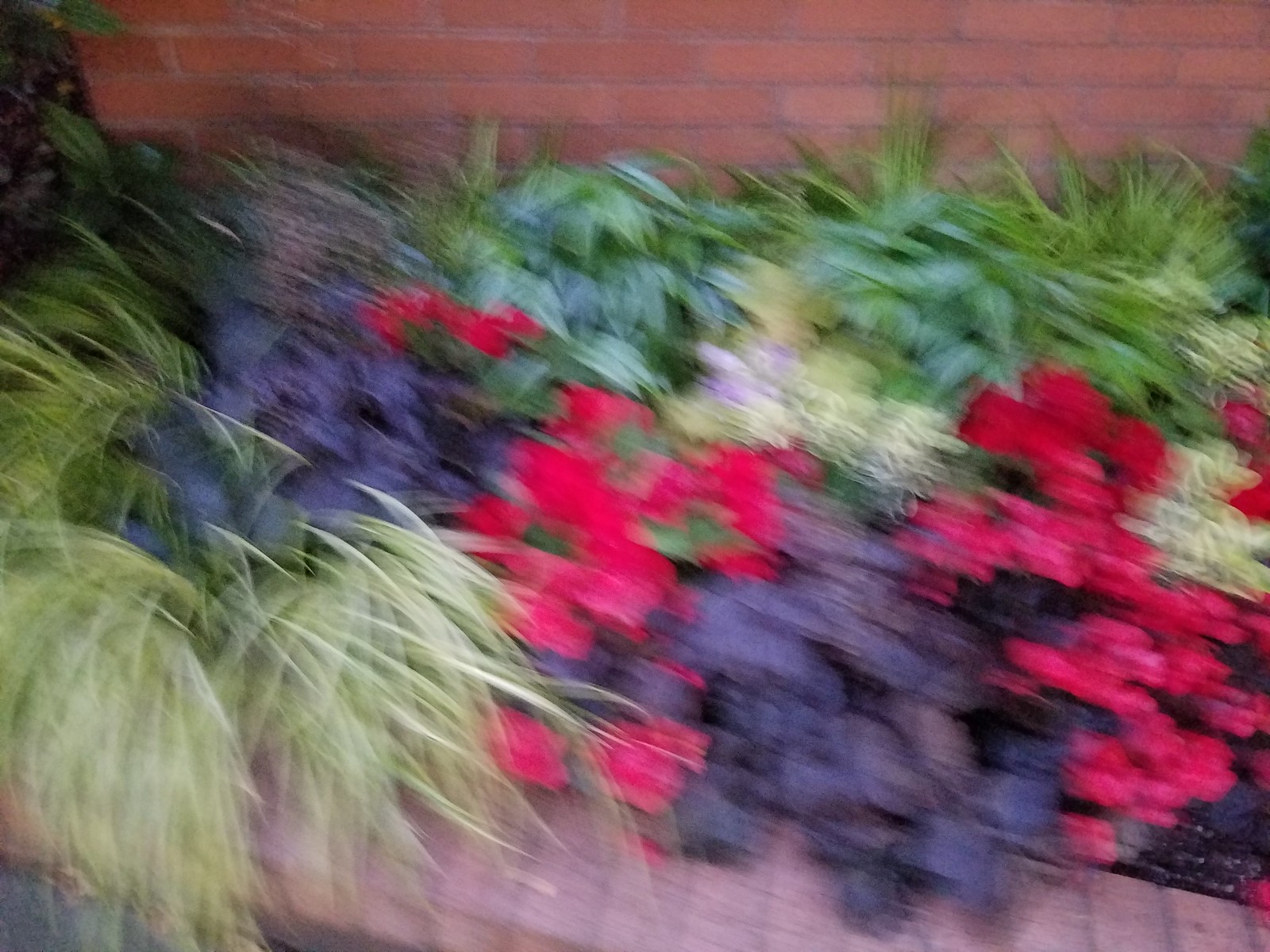In this image, a blurry and out-of-focus garden scene is captured. The garden features a variety of plants and flowers enclosed within a smaller, brown brick wall. Behind these plants is a larger brick wall, providing a backdrop to the scene. Despite the lack of sharpness, the foliage is distinguishable, exhibiting a range of colors including green, purple, bright red, and yellow. A small patch of dirt is visible in the bottom right corner, adding to the garden's natural appearance. The composition suggests a lush and vibrant garden area, albeit obscured by the poor focus of the photograph.